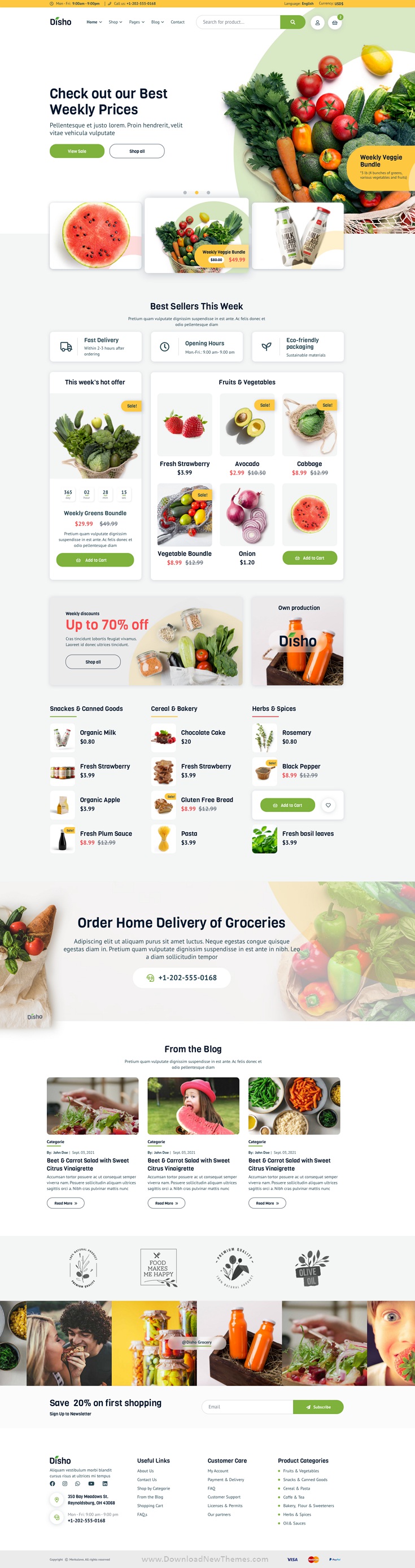The webpage features an array of food-related images and text. At the very top, there's a thin yellow line containing several lines of black text that are too small to decipher. Beneath this line, there's another set of black text with six words, followed by a white search bar with black text inside, adjacent to a green button labeled "OK" in white. Two small circular white icons are positioned to the right of these elements. Below, a prominent banner reads "Check out our best weekly prices," followed by two sentences in black text that are also unreadable.

Next is a green bar with white text, and below that is a white bar with black text. To the right, there's an image of a plate featuring an assortment of vegetables, including carrots, tomatoes, zucchini, broccoli, lemon, and cabbage. The bottom right-hand corner of this picture has a yellow tab with black text.

Below this, three white boxes each contain different images. The left box displays a close-up of a sliced watermelon with the pink flesh facing the camera. The middle box shows a similar plate of vegetables as previously described. The right box contains two glass bottles of milk, one with a green lid and the other with a red lid.

Further down, there's an image of a wicker basket filled with green leafy vegetables. Next to it, a container divides into three rows of images. The top left features two strawberries, the top middle shows a sliced avocado revealing its center, and the top right has another wicker basket with cabbage or lettuce. The middle left has a platter with different colored lemons and limes, the middle features purple onions, and the middle right shows a sliced watermelon with the pink flesh facing forward.

Beneath these images, red text on the left side announces "Up to 70% off," set alongside images of jars of honey and various vegetables. Also included is a picture of two glass bottles filled with an orange liquid. Below this, three sets of four images each, but these are too small to detail. The leftmost image depicts four stacked pictures, the middle follows the same arrangement, and the right contains two images plus a white box with a green bar featuring white text inside.

Moving down, there's an image of leafy vegetables followed by a bar with black text. On the left-hand side of this bar, a cloth bag filled with vegetables is shown, accompanied by the text "Order home delivery of groceries" in black. Below this, several sentences of black text are present.

The next section features three distinct pictures. The left image shows a right hand preparing food, underneath which is black text. The middle picture portrays a young Caucasian child with brown hair wearing a pink hat, consuming a large piece of watermelon, with black text included. The right image consists of several plates of chopped fruits or vegetables displayed on a table.

Lastly, a final row of images presents a partially cut-off image of bowls with cut fruits and vegetables on the left, a snapshot of a blonde girl and a brown-haired boy facing each other, both Caucasian, sharing a bite from the same item. Next is an image with a yellow backdrop showcasing several glass jars of canned fruits or vegetables. Adjacent to this is a picture with a white backdrop featuring a brown basket containing two glass bottles of an orange substance. Finally, there’s an image of prepared green fruit or vegetables, and to the far right, a stylized AI-generated image of a Caucasian boy eating something green.